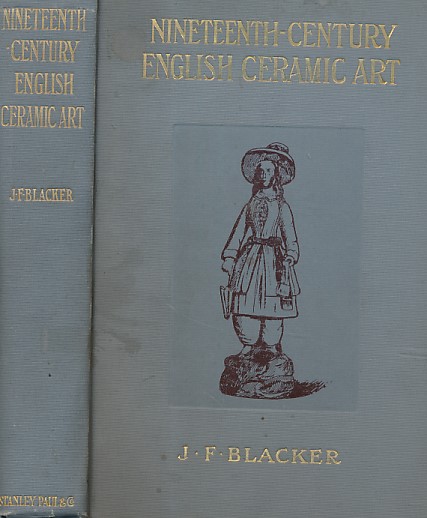This image features the cover and spine of an old, well-worn book with a canvas-like, medium-gray cover that has accumulated some dirt over time. The title, "19th Century English Ceramic Art," is prominently displayed at the top of the front cover in formal, gold-embossed lettering. Below the title, there is an illustration of a figure—possibly a pilgrim—wearing a long coat, long pants, and a large hat, though the figure’s gender is unclear. The author's name, J.F. Blacker, is inscribed in gold letters beneath the illustration. The spine of the book also bears the title and author’s name in the same gold-embossed style, along with the text "Stanley Plate and Company" at the bottom, indicating the book’s publisher.